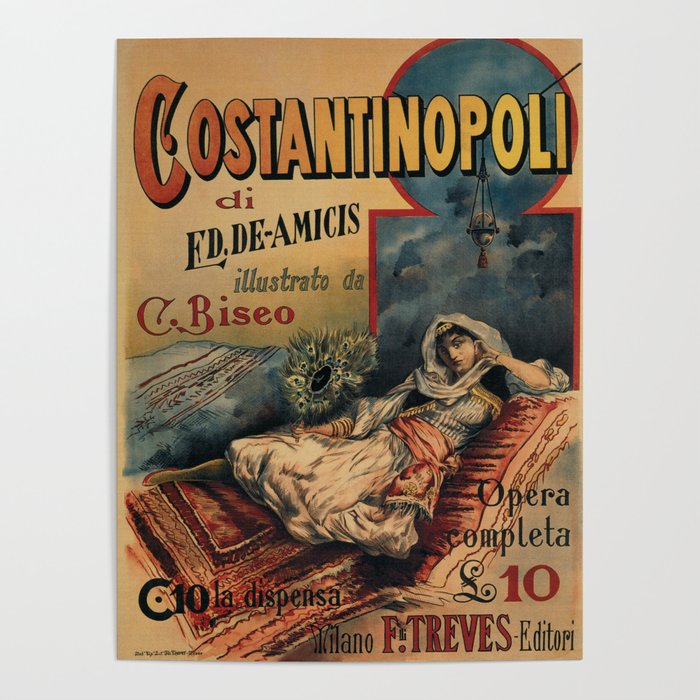The image depicts a vintage-style poster prominently displayed on a stark white wall. The poster itself has no border and is predominantly brown. At the top of the poster, the title "CONSTANTINOPOLI" is emblazoned in a distinctive 3D font, transitioning from orange to yellow, with a subtle black border around each letter. Below the title, text reads, "EDIAMICUS ILLUSTRATO DA C." The central illustration features a woman reclining elegantly on a chaise or cushion with red bedding, giving the appearance of an ornate chair. She dons a long gray gown and appears to resemble an Indian princess, her right elbow resting on a pillow and her hand thoughtfully touching her cheek. Near her right side, there is a decorative object adorned with peacock feathers. Beneath the illustration, additional text reads "OPERA COMPLETA X," with "La Dispensa" on the bottom left and "F. Trevis Editori" on the bottom right. The overall setting of the poster evokes a Middle Eastern ambiance, with a clear and well-lit photographic quality.